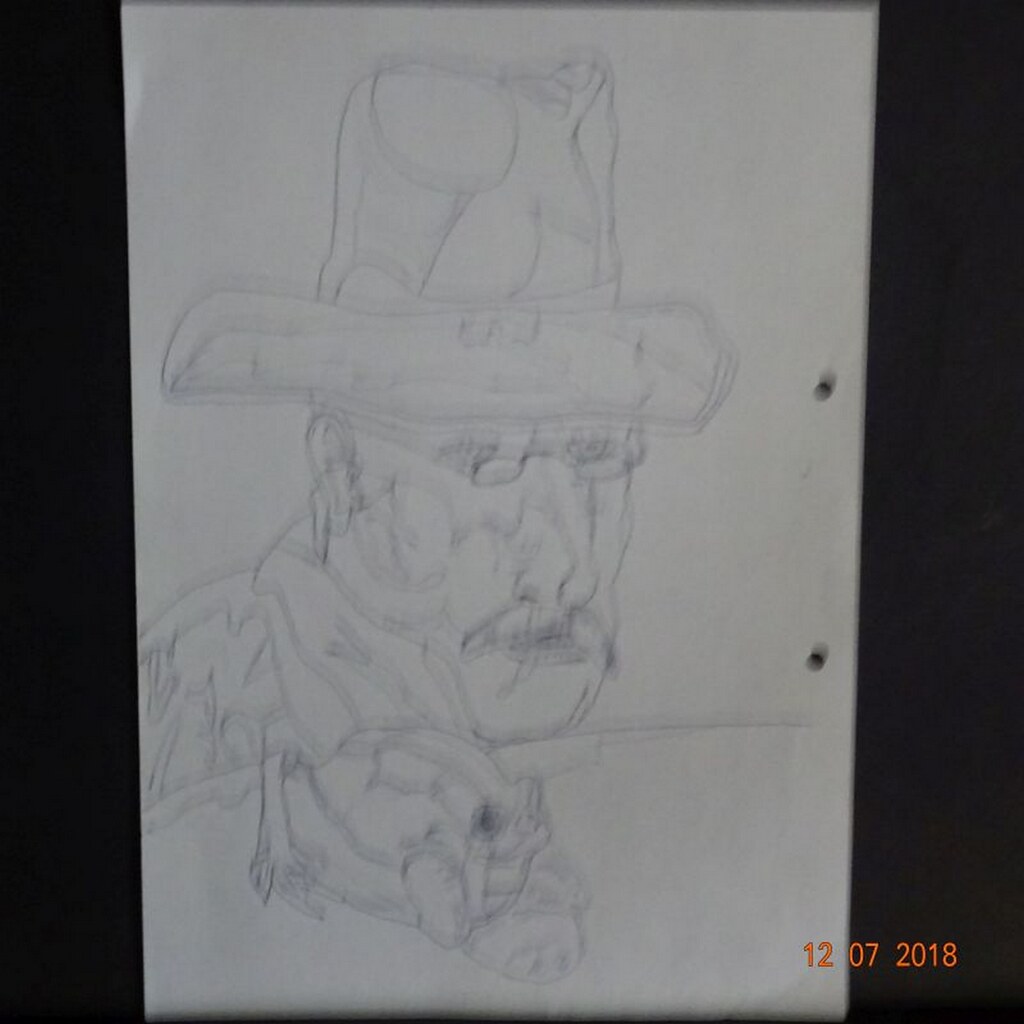This vertical photograph showcases a meticulously detailed drawing on a piece of paper, seemingly executed with a dark pen or pencil. At the bottom of the image, there's an orange-red date stamp reading "12-07-2018." The focal point of the drawing is a man, depicted in a slight side profile that highlights one ear. He is adorned with a hat, small glasses, and possibly a mustache. Perching on his shoulder and extending into the lower portion of the image is a peculiar creature. This creature is characterized by a leg with finger-like appendages and a prominent eyeball. The stark white background behind the man accentuates the details and intricacies of the drawing.